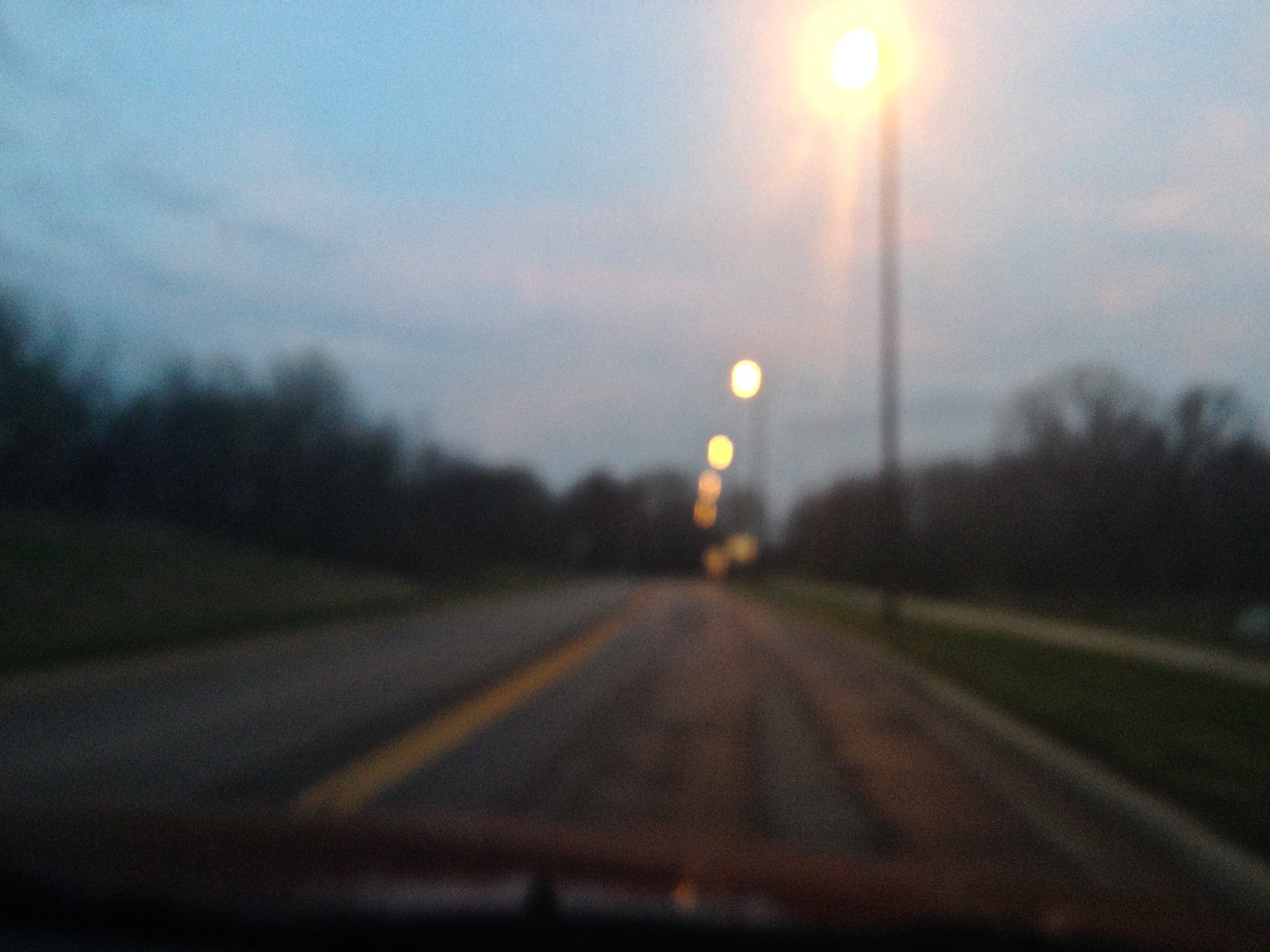This image captures a dimly lit, straight public road either at late evening or early night, with a distinct yellow centerline dividing the lanes. Grass flanks both sides of the road, providing a soft edge to the stark asphalt. In the background, the silhouettes of trees and bushy foliage are visible, adding a natural boundary to the scene. Overhead, several streetlights shine brightly, their intense glow obscuring the tops of the poles and casting a series of illuminated pools along the road. The overall atmosphere is one of quiet and solitude, with the bright streetlights punctuating the darkness.